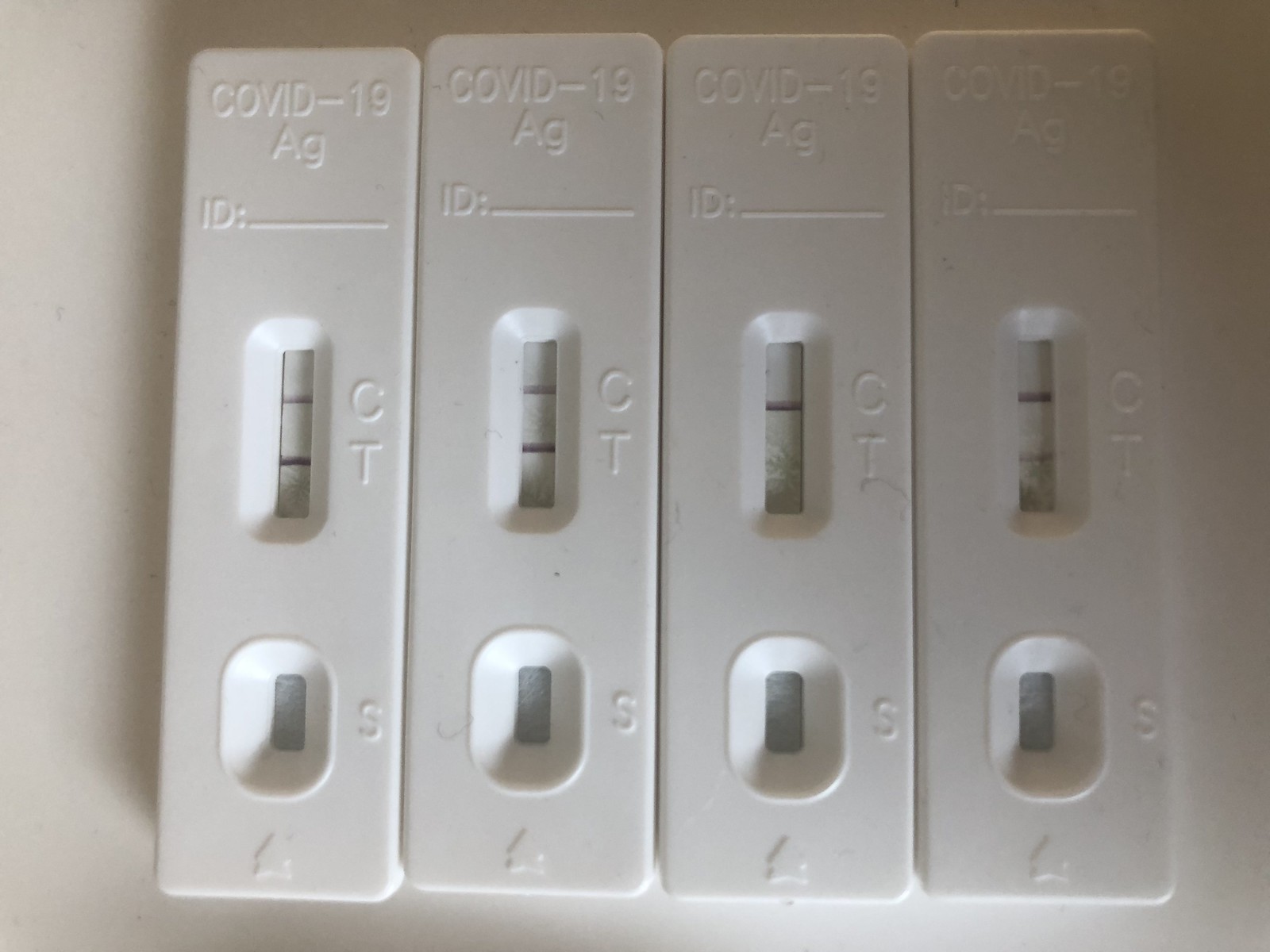This photo showcases four COVID-19 antigen test kits placed back-to-back on a white surface, likely illuminated by natural light given the softness of the shadows and absence of harsh yellow hues typical of artificial lighting. Each test kit, made of white plastic, features the label "COVID-19" engraved at the top, followed by "Ag" indicating it's an antigen test, an "ID" field with a blank line for personal information, and a display window that reveals the test results.

In the result window, the letters "C" and "T" are printed, where "C" represents the control line and "T" stands for the test result line. All four kits show a distinct purple line at "C," confirming the tests are functioning correctly. The first two tests clearly display two lines, indicating positive results for COVID-19. The third test shows a faint line at "T," suggesting a weak positive result, while the fourth test does not display a line at "T," signifying a negative result.

Below the result window, an "S" marks the location where the swab sample is to be placed, indicated by an arrow to guide users. The uniformity in design and clear labeling aims to ensure user-friendly operation and accurate interpretation of test results.